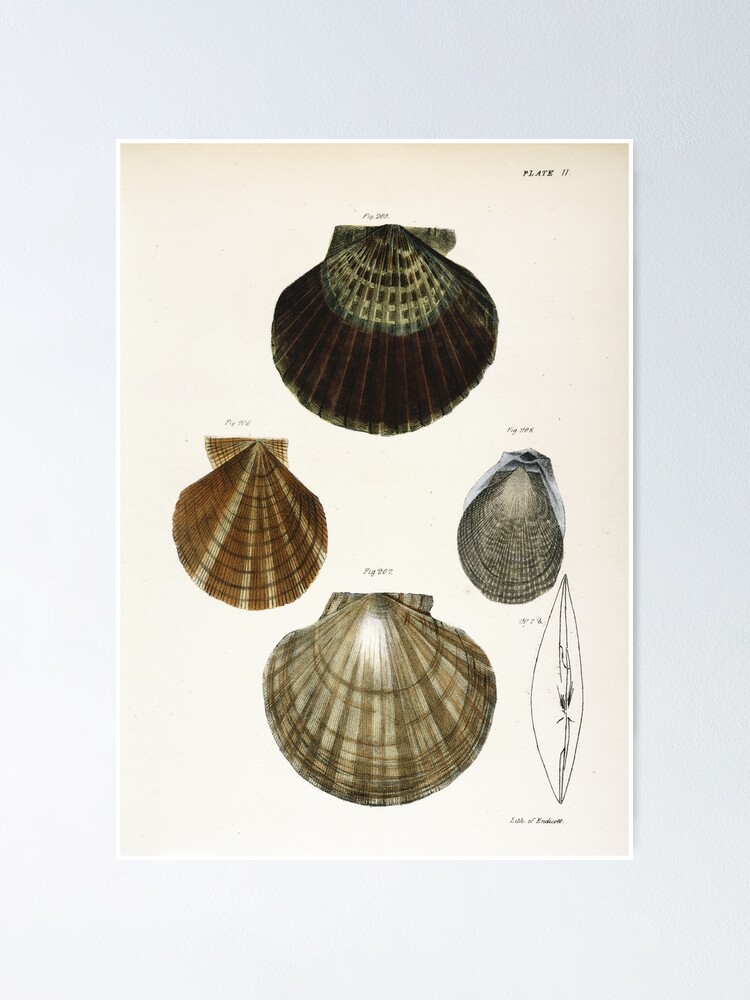This is a detailed scientific diagram on slightly yellowed paper with darkened edges, depicting four different types of clamshells, observed from a top-down perspective. Each clamshell varies in color and pattern: the top shell, labeled "Figure 265" and situated under the heading "Plate 11," is dark brown with light gray-blue concentric layers towards its narrow end. The left middle shell, marked "Figure 106," is light brown featuring diagonal white stripes, while the right middle shell, labeled "Figure 105," is predominantly gray with fine white pinstripes. The bottom shell, identified as "Figure 207," exhibits a tan background with brown stripes and additional black and gray lines accentuating its outer edges. All clams are positioned with their narrow ends pointing downward. Additionally, a black and white side profile drawing of a clamshell can be seen at the bottom right corner of the page.